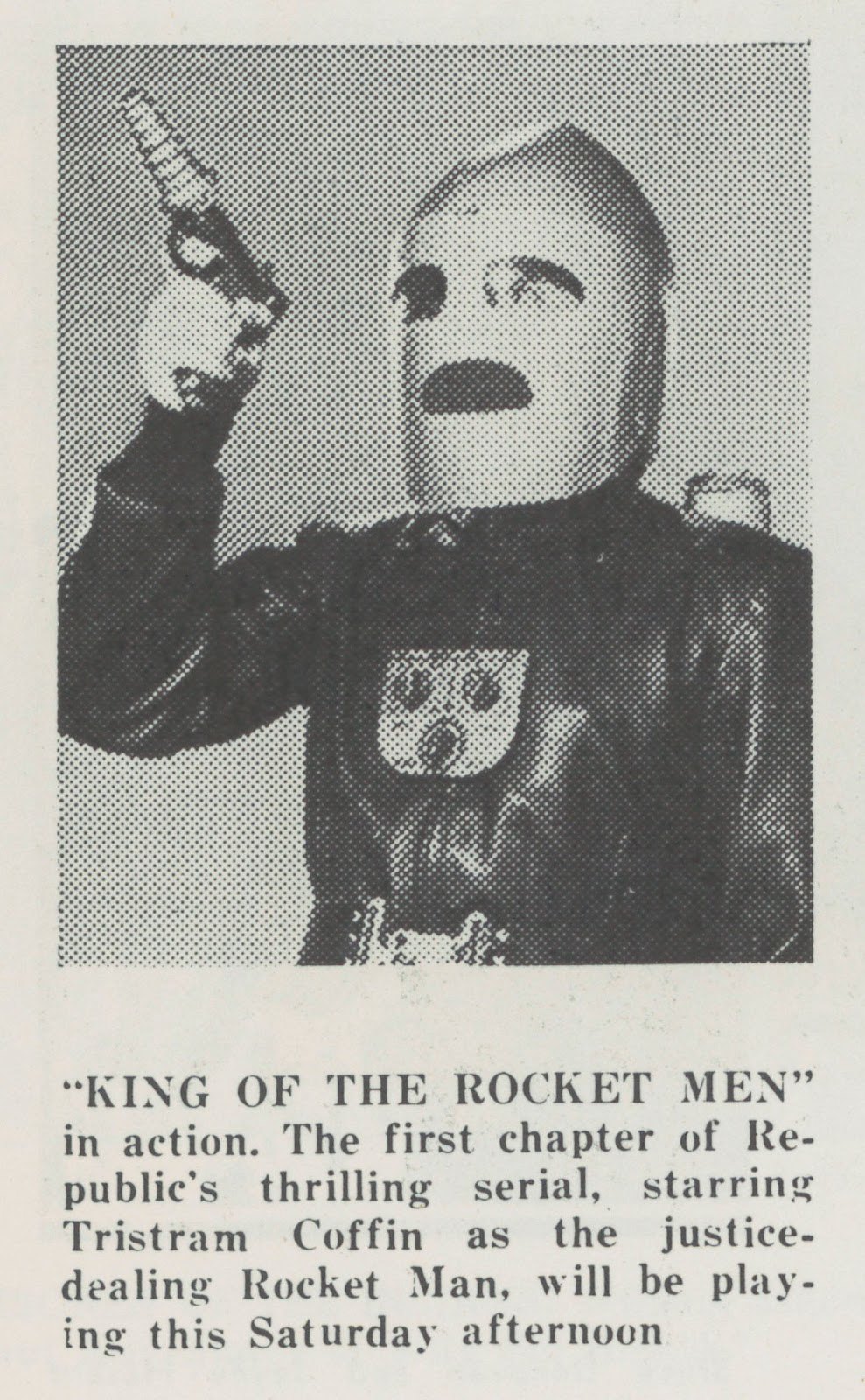The image appears on a light blue background. The photograph, which occupies the top part of the image, is black and white and has a grainy appearance, suggesting it is quite old. The photograph features a man wearing a dark jacket adorned with dials on his chest, holding a ray gun that he points towards the upper left corner. He is also equipped with a helmet. Below the photograph, in dark gray letters, the caption reads:

"King of the Rocket Men - In action! The first chapter of Republic's thrilling serial starring Tristram Coffin as the justice-dealing Rocket Man will be playing this Saturday afternoon."